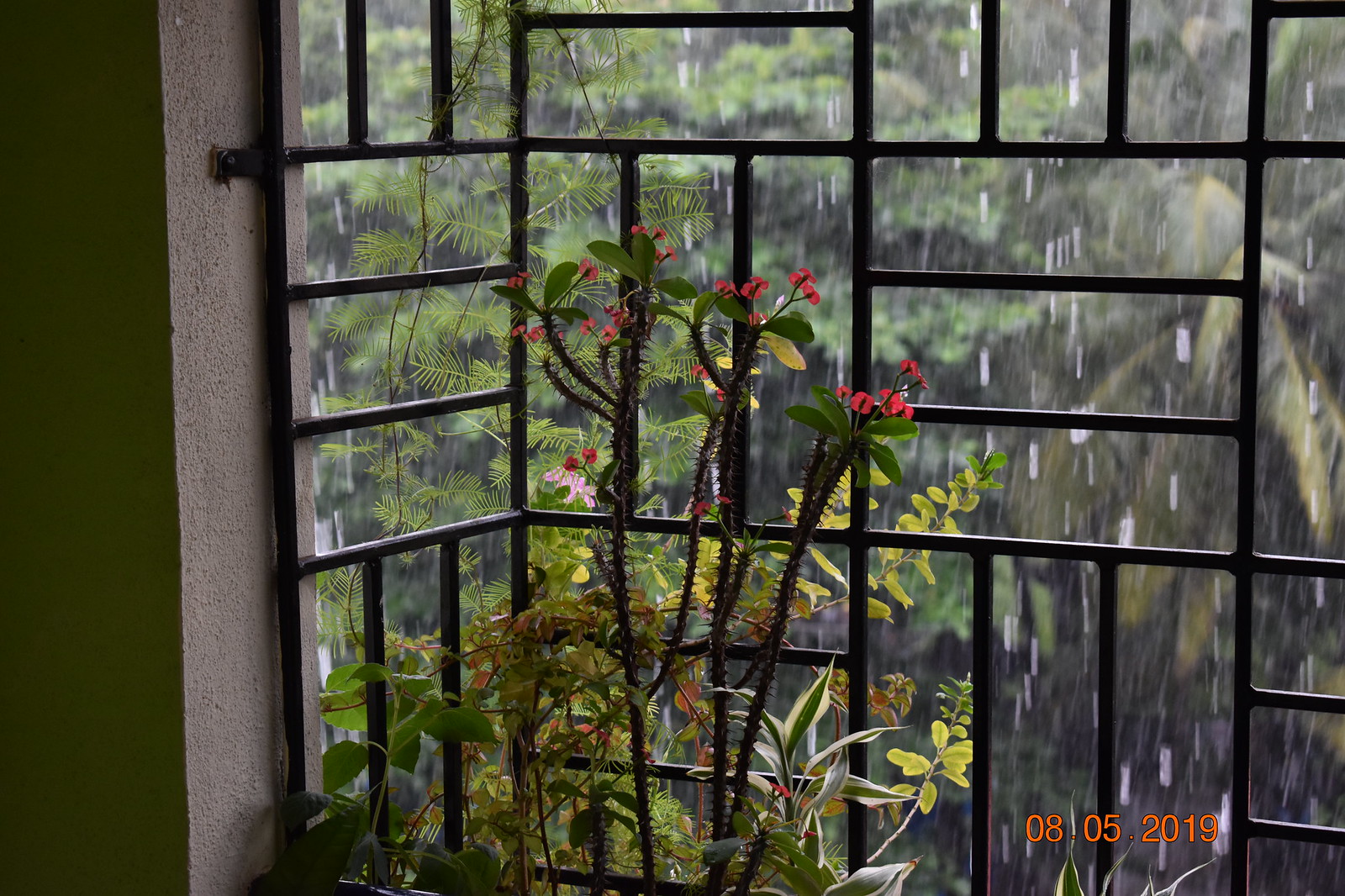The detailed image captures a scene viewed through a distinct window, presumably from inside a residence. The window is framed with brown metal bars arranged in various shapes, resembling a cage-like structure. Just inside the window, there is a plant with long stems adorned with small, vivid red flowers, which is the main focus of the image. Beyond the bars, a lush green garden or forest area is visible, albeit blurred, indicating rainfall as blurred raindrops cascade down. Additionally, to the left side of the image, there is a beige concrete wall visible inside the space. The entire scene is well-illuminated with natural light, suggesting the photograph was taken during daytime. The image is dated 08-05-2019, with the date stamped in orange in the lower right corner.